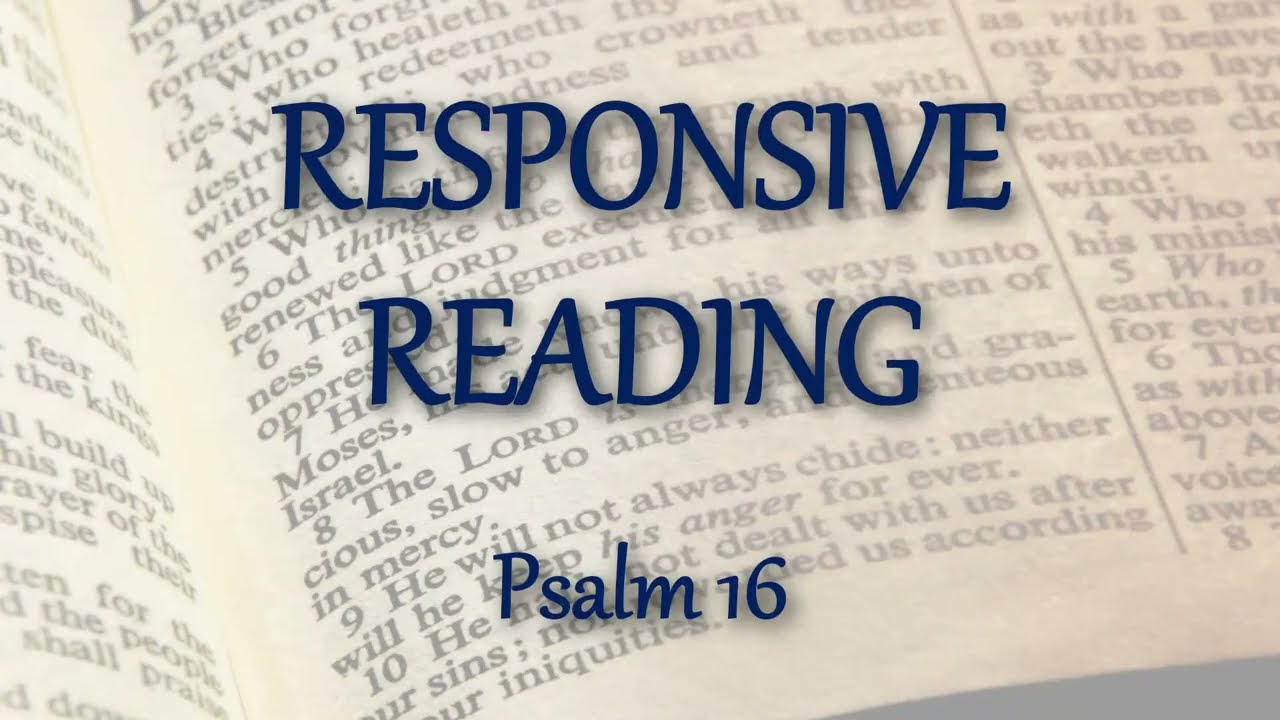A zoomed-in perspective of an open Bible dominates the center of this image, with about 75% of the frame dedicated to a single page. This page is bisected vertically, and the photograph focuses on one of the halves. The page is slightly blurred and faded into the background, creating an out-of-focus effect that diminishes the clarity of the black text on the page. Superimposed over the center of the image, in large, bold, uppercase black letters, are the words "RESPONSIVE READING." Below this header, in smaller yet prominent blue letters, is the title "Psalm 16." The open Bible reveals fragments of the psalm, starting from about section 2 and continuing through section 10, although some of these sections are partially cut off due to the zoomed-in nature of the shot. The overall effect is a striking contrast between the faded scripture page and the vivid superimposed text, clearly distinguishing the religious context of the photograph.